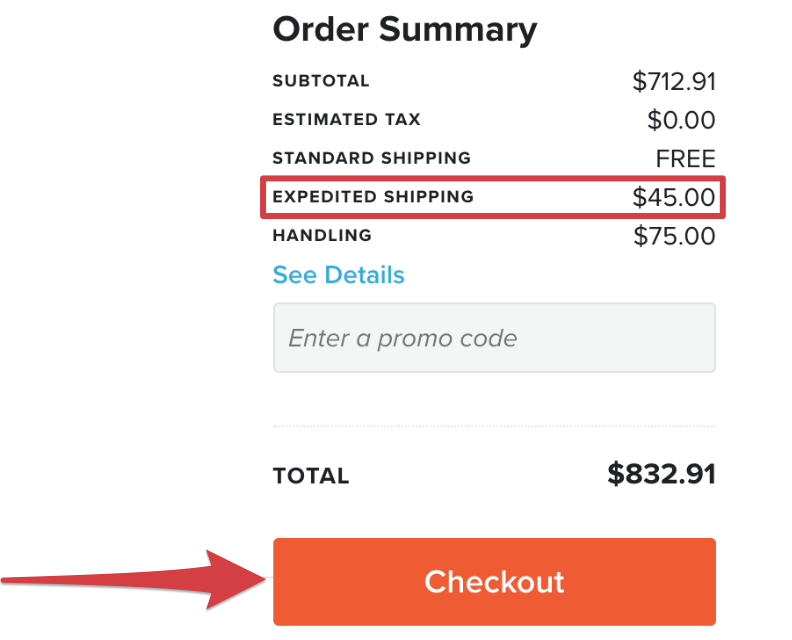The following is a close-up screenshot of an order summary. At the top of the screen, bold text clearly states, "Order Summary." The subtotal is prominently displayed in smaller yet bold text as "$712.91." Below this, "Estimated Tax" is also in all caps and bold, with the amount listed as "$0." 

"Standard Shipping" is marked as free, while "Expedited Shipping" is highlighted with a thick red border and costs "$45." Beneath that, "Handling" is detailed with a fee of "$75." A clickable "See Details" link in lighter blue text provides further information if needed.

A pale gray text box prompts, "Enter a Promo Code," followed by a dotted gray line. The total amount due is displayed in bold at "$832.91." 

At the bottom of the screenshot, a large red-orange button with white text, spanning the entire width of the screen, reads "Checkout." A large arrow is pointing towards this checkout button.